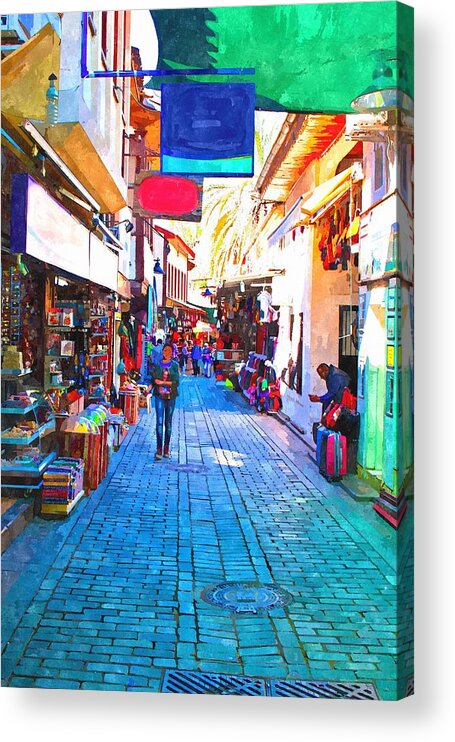The canvas painting depicts a bustling bazaar or shopping district filled with colorful vibrancy and dynamic elements. The scene is set on a brick and cobblestone street that runs between two rows of small shops teeming with souvenirs, trinkets, and various goods, from backpacks and suitcases to food items. Above the street hangs a bright green canopy, through which the sun shines, casting a green-tinted light over the scene below. Vivid reds, blues, yellows, and oranges saturate the image, enhancing the lively atmosphere.

Several individuals populate the bazaar, including a young woman in blue jeans and a blue jacket walking toward the foreground, carrying something in her hands. To the right, a gentleman sits next to his store, surrounded by his merchandise, appearing deep in thought. Further along the sidewalk, another man stands in an alcove decorated with green and yellow hues, checking his phone beside his suitcase. A notable feature in the background is a blown-out palm tree, adding to the sunny and warm ambiance of the scene.

Despite the indistinct and blurred facial features of the people, their actions and attire contribute to the overall energetic and vivid depiction of a foreign marketplace, brimming with life and color.